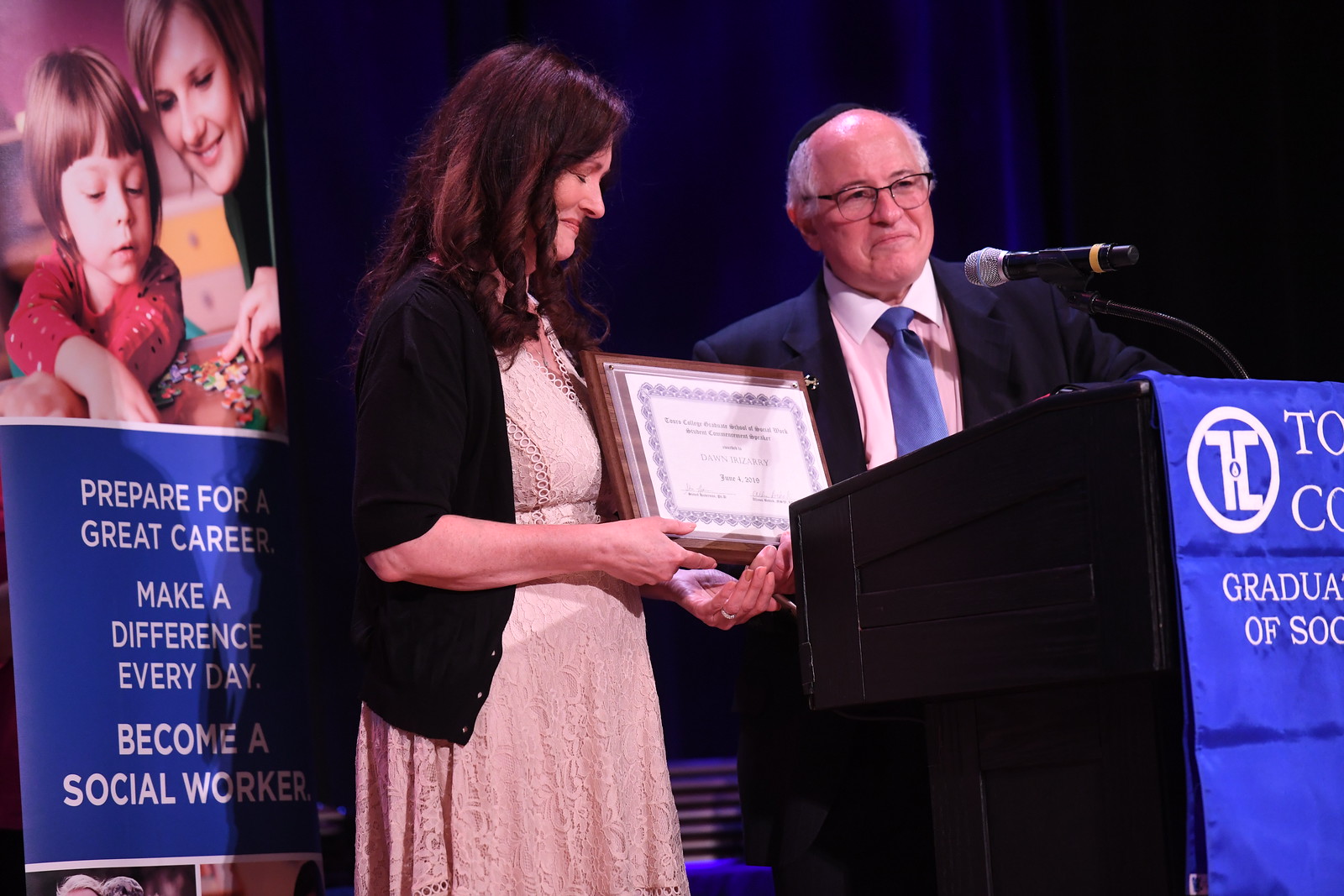In this photograph, set at an indoor award ceremony, two central figures stand behind a black lectern adorned with a blue banner and a microphone. The backdrop is a navy blue curtain, and a prominent sign features a picture of a woman and a baby with the words: "Prepare for a great career, make a difference every day, become a social worker."

The woman, a white individual with brown hair, is wearing a long cream-colored dress paired with a dark sweater. She is receiving an award mounted on a wooden plaque and smiles warmly at it. To her side, an older man with a balding head, gray hair on the sides, and glasses, dressed in a dark suit with a white shirt and blue tie, stands attentively. He is positioned slightly to the left of the microphone, looking out into the audience. The overall setting suggests a celebration or recognition event, likely connected to a graduate school or a career day focusing on social work.